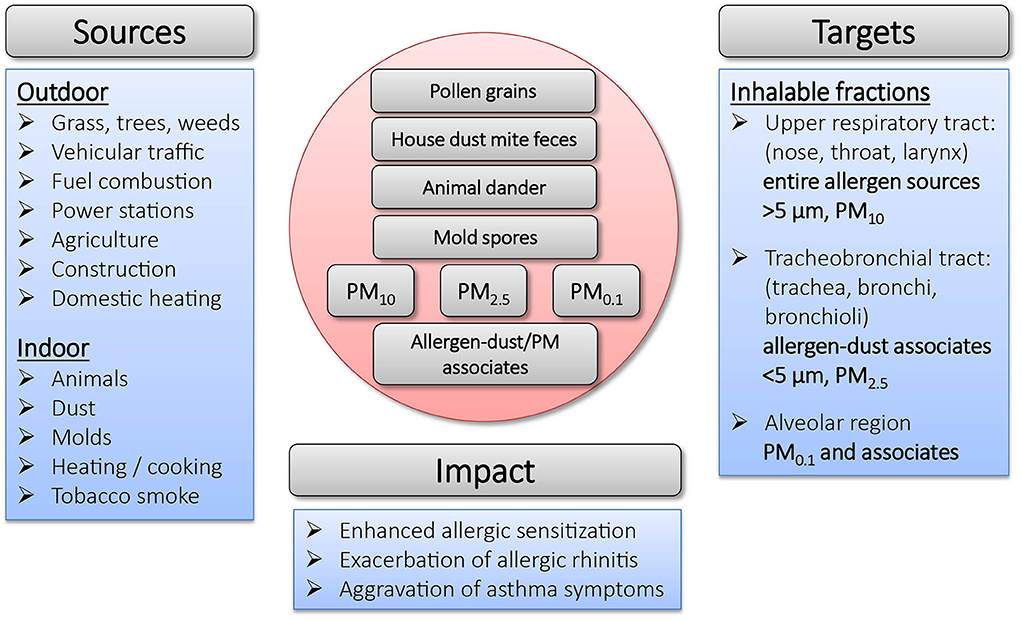This image features a detailed diagram about the sources, impacts, and targets of allergens. 

In the upper left, a gray rectangular area labeled "Sources" identifies various contributors to allergens. Outdoor sources include grass, trees, weeds, vehicular traffic, fuel combustion, power stations, agriculture, and construction. Indoor sources encompass animals, dust, mold, heating, cooking, and tobacco smoke. 

At the center of the diagram, a pink circle lists specific allergens, including pollen grains, house dust mite feces, animal dander, mold spores, PM10, PM2.5, PM0.1, and allergen dust/particulate matter associates.

On the right, another gray rectangular area labeled "Targets" outlines the affected bodily regions, specifying the inhalable fractions such as the upper respiratory tract (nose, throat, and larynx), tracheal and bronchial tracts, and the alveolar region.

At the bottom, a blue rectangular section titled "Impact" describes the health effects of these allergens, including enhanced allergic sensitization, exacerbation of allergic rhinitis, and aggravation of asthma symptoms. This comprehensive diagram effectively illustrates the intricate relationships between allergen sources, their specific manifestations, targets within the respiratory system, and overall health impacts.